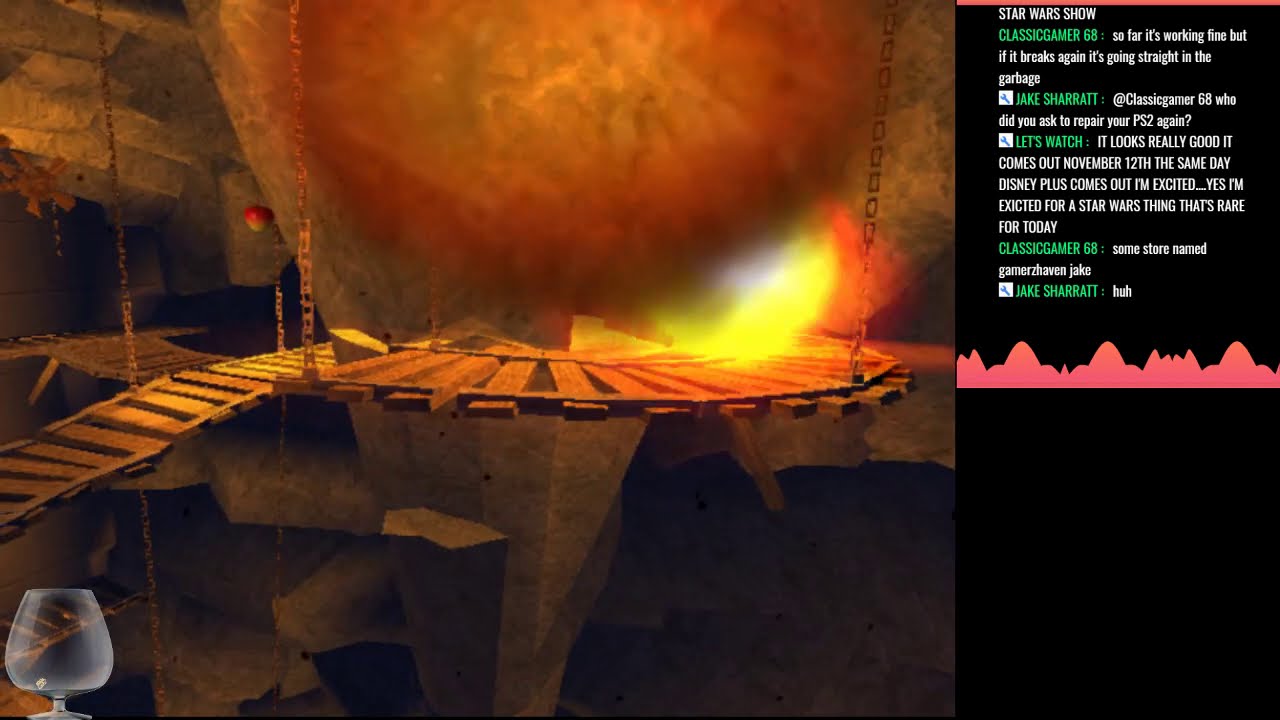The image appears to be a screenshot from a video game, possibly from a stream on a platform like Twitch, given the chat overlay on the right side. The scene is set in what looks like a mine shaft or underground encampment, characterized by stone walls and outcroppings. Central to the image is a large, suspended wooden bridge composed of wooden planks and supported by rusted black chains, creating a mix of straight and rounded sections. A vibrant flame is visible on one side of the bridge, adding an element of danger and warmth to the setting. The color palette includes earthy browns for the wood and stone, with bright yellow and orange accents from the fire. On the lower left corner of the image, there's an overlay featuring a clear wine glass logo, adding a unique watermark-like detail. The right side of the screenshot is dominated by a black chat column, featuring usernames in green and messages in white text, with a red line graph visible beneath them. At the top of this chat column, the text "Star Wars Show" indicates what the users might be discussing or the name of the stream. The overall style of the game resembles classic PlayStation-era graphics, with floating red and yellow apples reminiscent of a game like Crash Bandicoot, adding a nostalgic touch to the modern streaming interface.